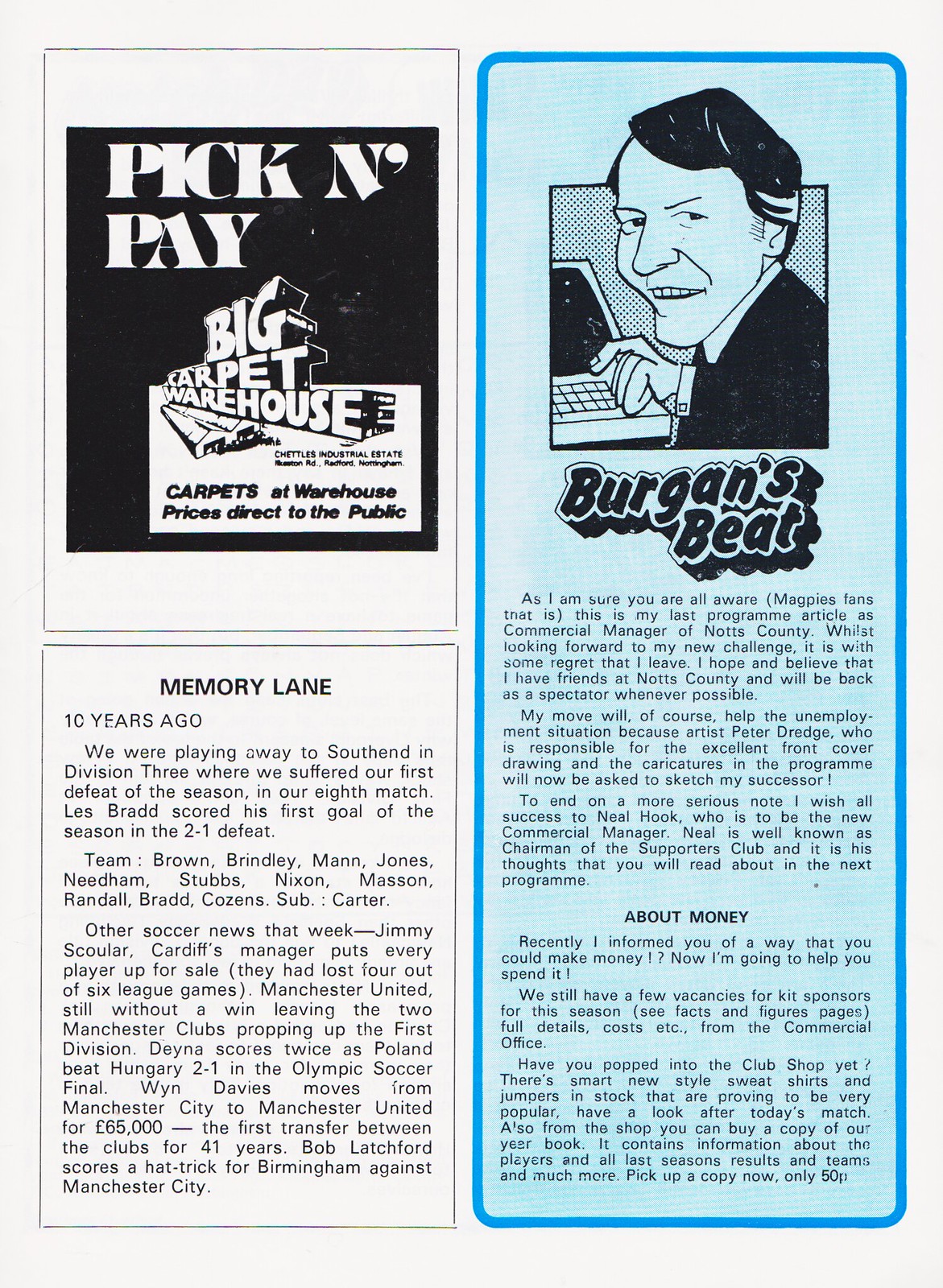The image is divided into three distinct sections. On the left, set against a black background, there is an advertisement for "Pick and Pay Big Carpet Warehouse" featuring text that highlights "carpets at warehouse prices direct to the public" alongside a drawing of two warehouses. Below this ad is a segment titled "Memory Lane," which details a nostalgic sports article about a match 10 years ago where a team suffered their first defeat of the season against South End in Division 3, with Les Bradd scoring his first goal in the 2-1 loss. On the right side, against a blue background with a black border, is an advertisement for "Bergen's Beat," presented in black lettering. This side of the image also seems to contain an article, framed with a blue border, contributing to the overall look of a magazine page composed of ads and articles.